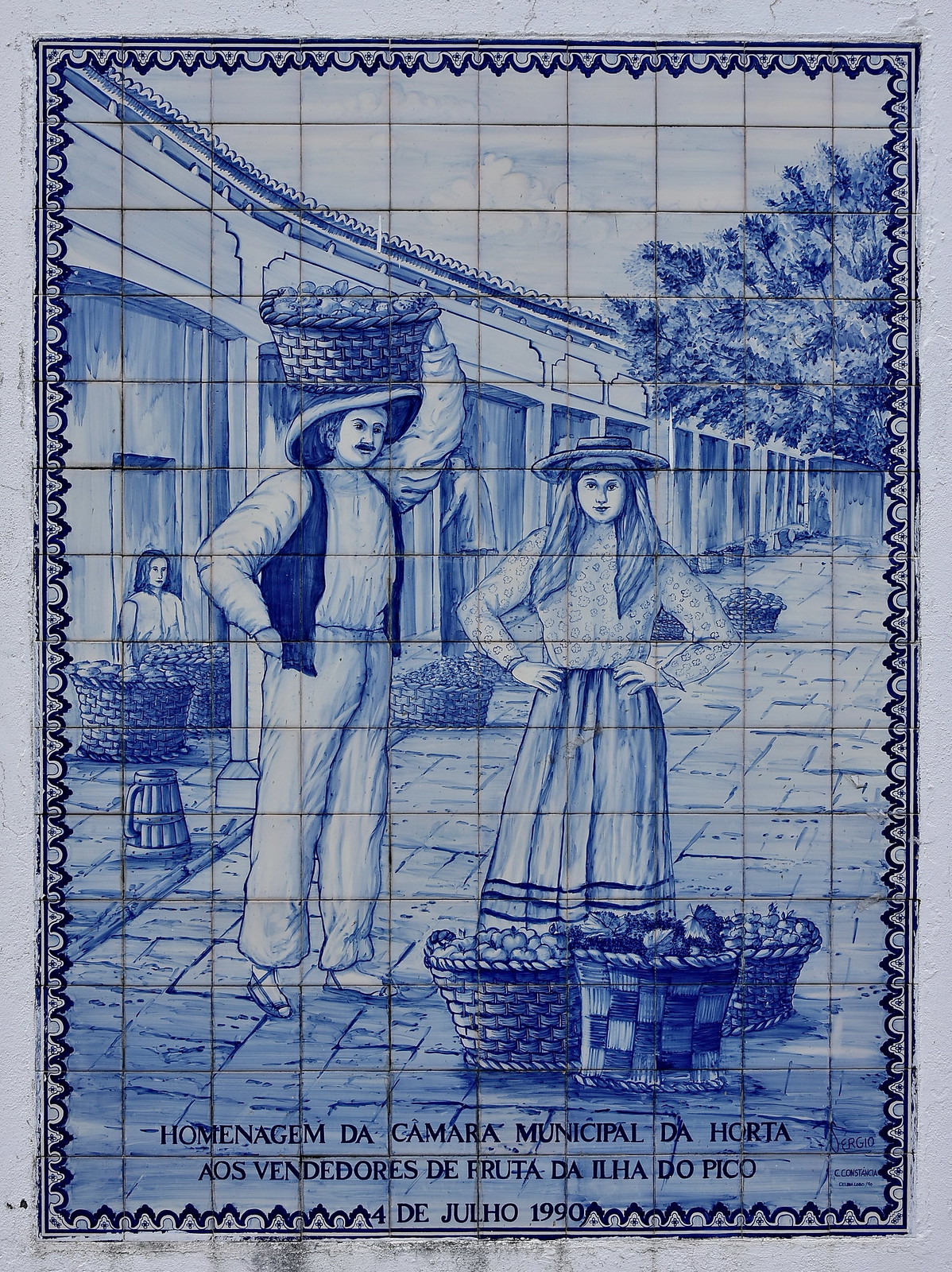The photograph showcases a detailed tile work featuring a man and a woman standing on a stone or brick road. The entire image is rendered in shades of blue, black, and white, and is segmented by grid-like lines indicative of individual tiles. The man is depicted wearing flowing pants, sandals, and a white shirt with a dark vest. He balances a basket of produce on his head with one arm while his other hand is in his pocket. The woman beside him is dressed in a full blouse and a long skirt with lines at the bottom. She wears a long hat atop a bandana that flows down, and her hands rest on her hips. In front of them are three larger baskets containing a mix of fruit and bread. The background includes a tree on the top right side and a large structure on the left. At the bottom of the tile work, there is an inscription in a foreign language, possibly Spanish, reading "Homologen da Camera Municipal da Horia Es Vendores de Fruta de la Libago de Julio 1990," suggesting the scene depicts fruit sellers in July 1990.